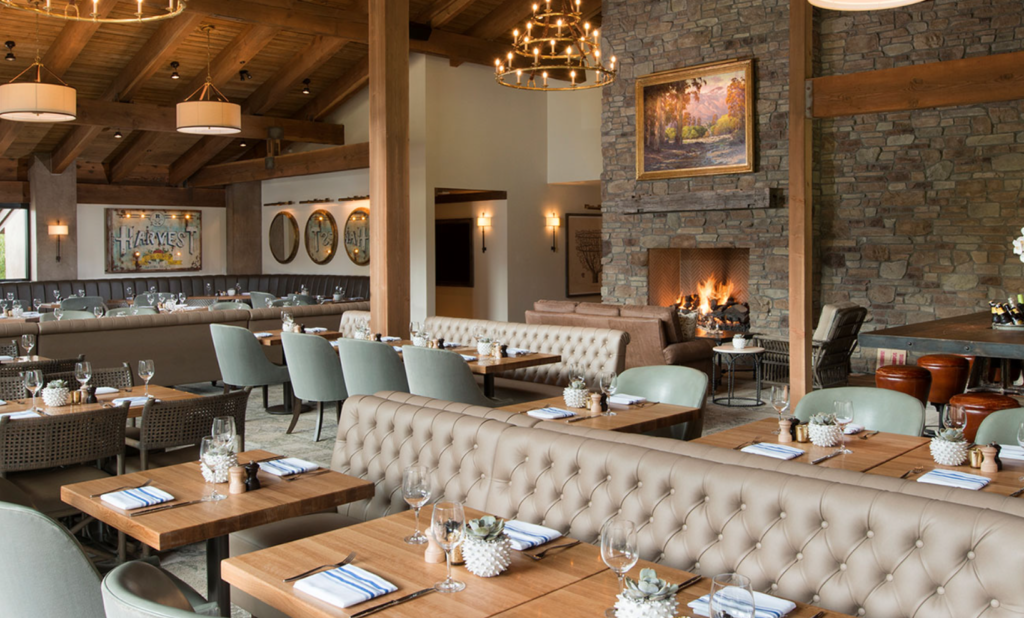The image depicts the spacious interior of a restaurant before its opening, with no people present. The dining area features a mix of light wooden standalone tables and cushioned booths. The booths have a light brown upholstery, whereas the standalone tables are paired with light green chairs. Each table is meticulously set with napkins, silverware, and glasses, accompanied by decorative centerpieces that add a touch of elegance. The restaurant exudes a cozy, woodsy ambiance, reminiscent of a fancy cabin, highlighted by wooden beams and a cobbled stone wall in the background. The wall behind the booths showcases an inviting, lit fireplace, reinforcing the warm atmosphere. White walls are visible to the left, adorned with various pieces of art. Illuminating the space, chandeliers and minimalist lamps hang from the ceiling, enhancing the sophisticated yet rustic charm. Additionally, a large poster on the far left reads "Harvest," adding to the restaurant's theme. The scene also includes notable details like a leather couch, light switches, and wooden pillars that further contribute to the overall aesthetic of this refined dining spot.